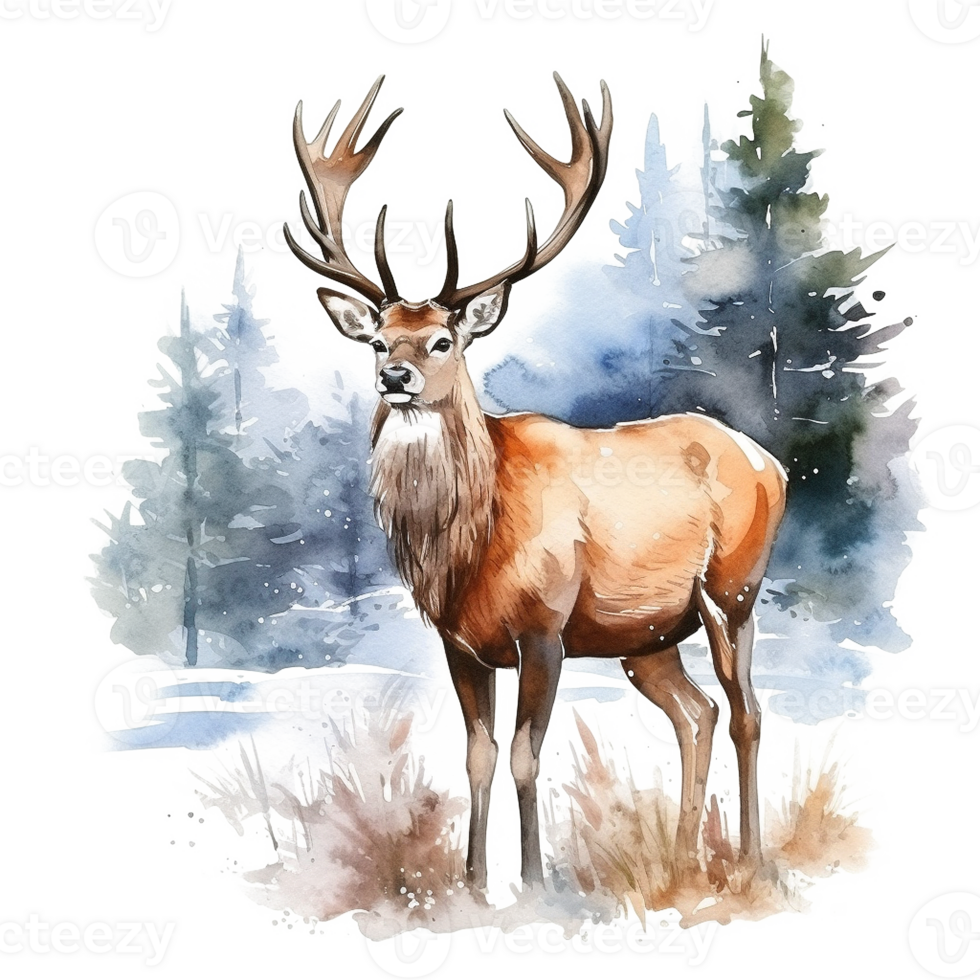This painting, set outdoors in the soft natural light of winter, features a majestic buck deer standing in a snow-covered landscape. The buck has a striking appearance with his tall, dark brown legs, a lighter brown body, and a thick, white beard around his neck, which is unique and adds to his grandeur. His dark eyes and large, impressive antlers draw immediate attention. The ground around him is blanketed in snow, with tufts of brown grass peeking through. The background, which gives an impressionistic feel, showcases pine trees with a bluish hue, some of which are blurred to add depth. Snow appears to be gently falling, adding to the serene, cold atmosphere. The sky above is a bright white, further emphasizing the winter setting. There's a hint of a pathway to the left of the deer, possibly a snow-covered road with a few blue-tinged puddles, contributing to the scene's tranquil but chilly ambiance.